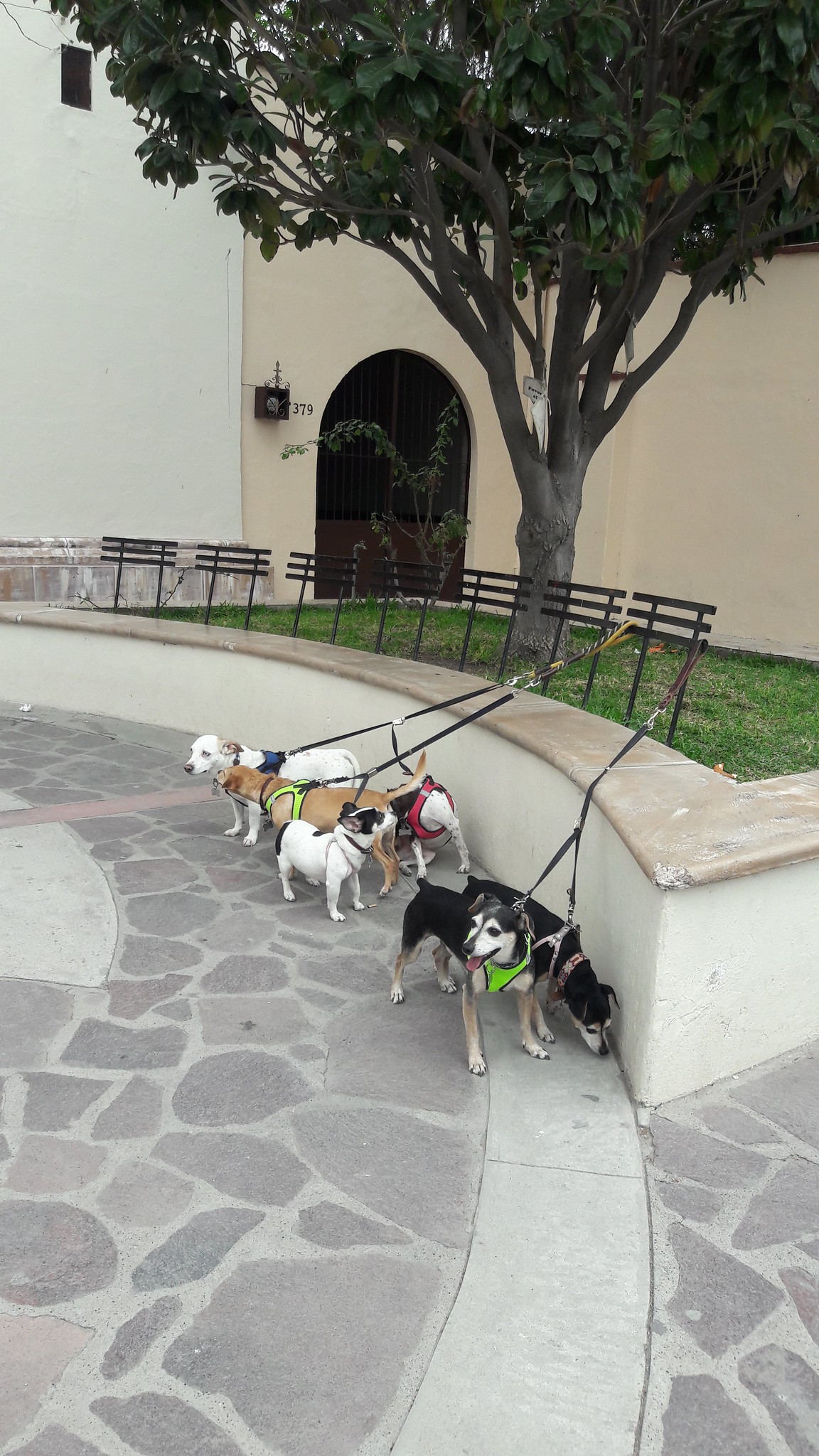In this outdoor photograph, there are six small to medium-sized dogs, each tethered by black leashes to a series of black post-like structures, likely designed for this purpose. The ground they are standing on is a circular, rocky pavement composed of flat stones in various shades of gray. The dogs are a mix of colors: two black, three white, and one light brown. Notably, one of the white dogs' head is obscured by the light brown dog standing in front of it. In the background is a patch of grass and a single tree lush with green leaves. Further behind, there's a beige concrete building, with only a portion of its front visible. The scene is framed by the surrounding elements which give it a courtyard feel, potentially Spanish in style, enhancing the picturesque, rustic ambiance.